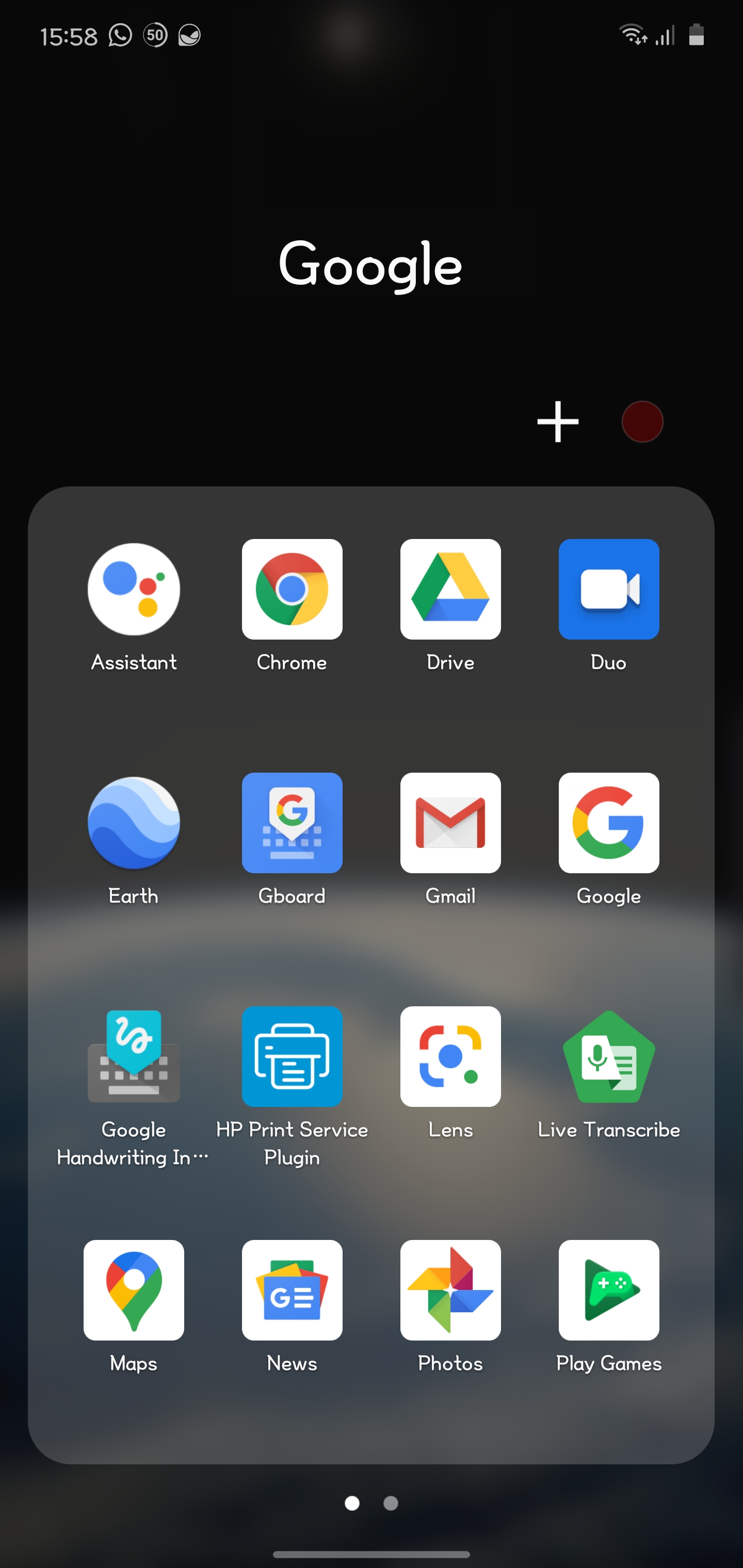This image showcases the Google homepage displayed on a black background, with the iconic "Google" wordmark prominently featured in white text at the top, occupying roughly the upper third of the screen. Below the logo, there is a grid of sixteen icons arranged in four rows and four columns, providing easy access to various Google services and applications.

- **First Row:**
  - **Assistant:** A blue, red, and yellow series of circles inside a larger white circle.
  - **Chrome:** The recognizable Chrome browser icon.
  - **Drive:** The triangular Drive icon colored in green, yellow, and blue.
  - **Duo:** A white camera icon on a blue background.

- **Second Row:**
  - **Earth:** Depicted by a blue and white globe.
  - **Gboard:** An icon symbolizing the Gboard keyboard app.
  - **Gmail:** An envelope icon, representing the Gmail email service.
  - **Google:** A stylized multicolored "G".

- **Third Row:**
  - **Google Handwriting Input:** The visible portion of the icon suggests a drawing tool.
  - **HP Print Service Plugin:** An icon displaying a printer.
  - **Google Lens:** Represented by a blue circle with multicolored brackets around it.
  - **Live Transcribe:** An icon featuring a microphone overlaying a document.

- **Fourth Row:**
  - **Google Maps:** Represented by a location pin icon.
  - **Google News:** An icon representing breaking news.
  - **Google Photos:** The multicolored pinwheel icon.
  - **Play Games:** An icon depicting a game controller.

Each icon is easily distinguishable, offering quick access to Google's vast array of applications and services directly from the home page.